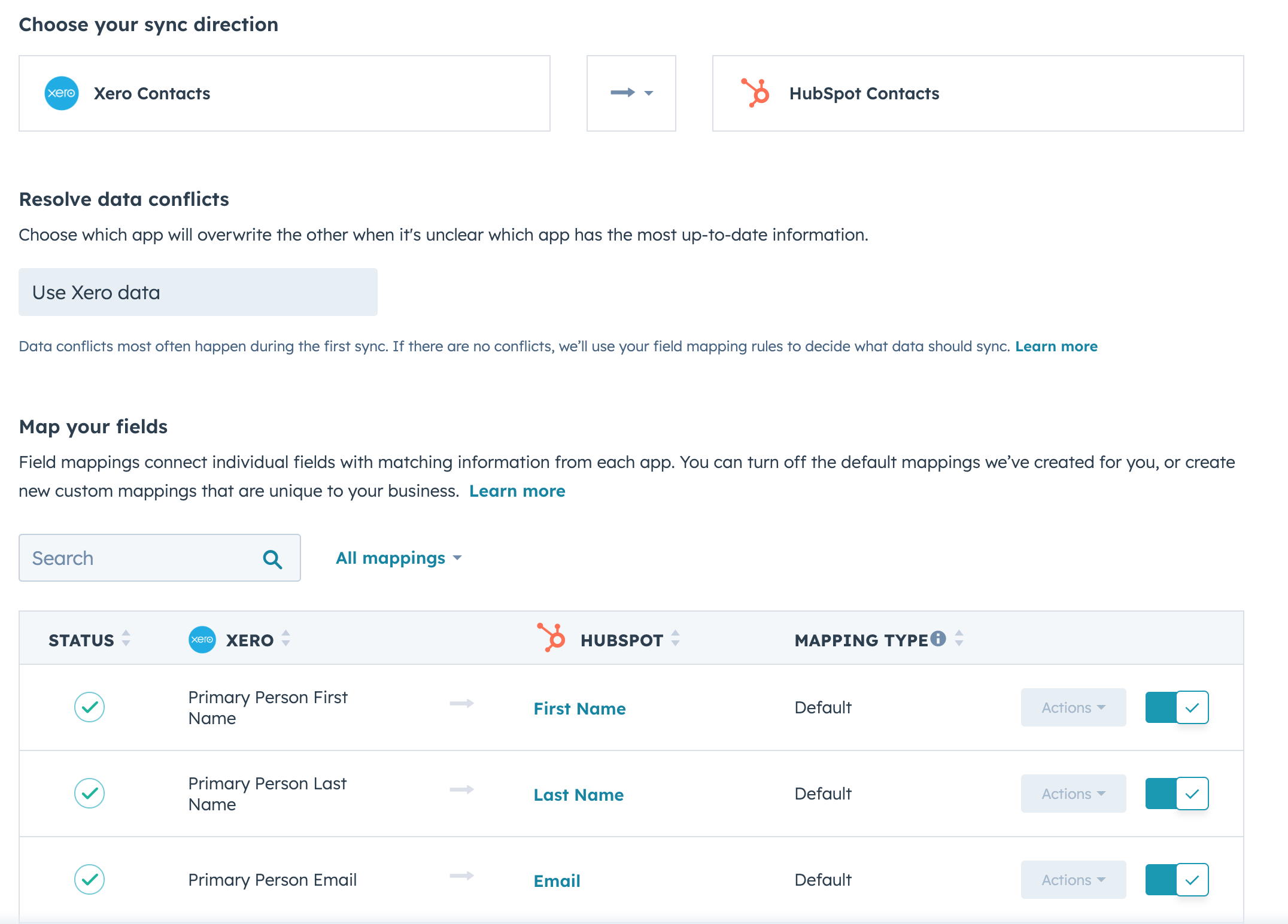**Screenshot of App Settings: Sync and Data Conflict Resolution**

The image is a screenshot of an app's settings, featuring a clean, white background. Positioned prominently at the top left corner, the heading "Choose Your Sync Direction" is displayed in bold black font. 

Immediately below, a rectangular section reads "Xero Contacts," where "Xero" is spelled with an 'X'. To the right of this section, there is a small gray box containing a right-pointing arrow. Further to the right, another rectangle is labeled "HubSpot Contacts."

Underneath this part, a section titled "Resolve Data Conflicts" is presented. The text beneath this heading explains, "Choose which app will overwrite the other when it's unclear which has the most up-to-date information."

Following is a gray rectangle stating "Use Xero Data" in black font, again spelling "Xero" with an 'X'. Positioned below, in a subtler gray font, it is noted that "Data conflicts most often happen during the first sync." Additionally, if there are no conflicts, your designated field mapping rules will determine the data that should sync. There is also a clickable "Learn more" link highlighted in blue.

The final section of the screenshot is titled "Map Your Fields," describing how field mappings connect individual fields with matching information from each app. Users have the option to turn off the default mappings that have been pre-configured for them.